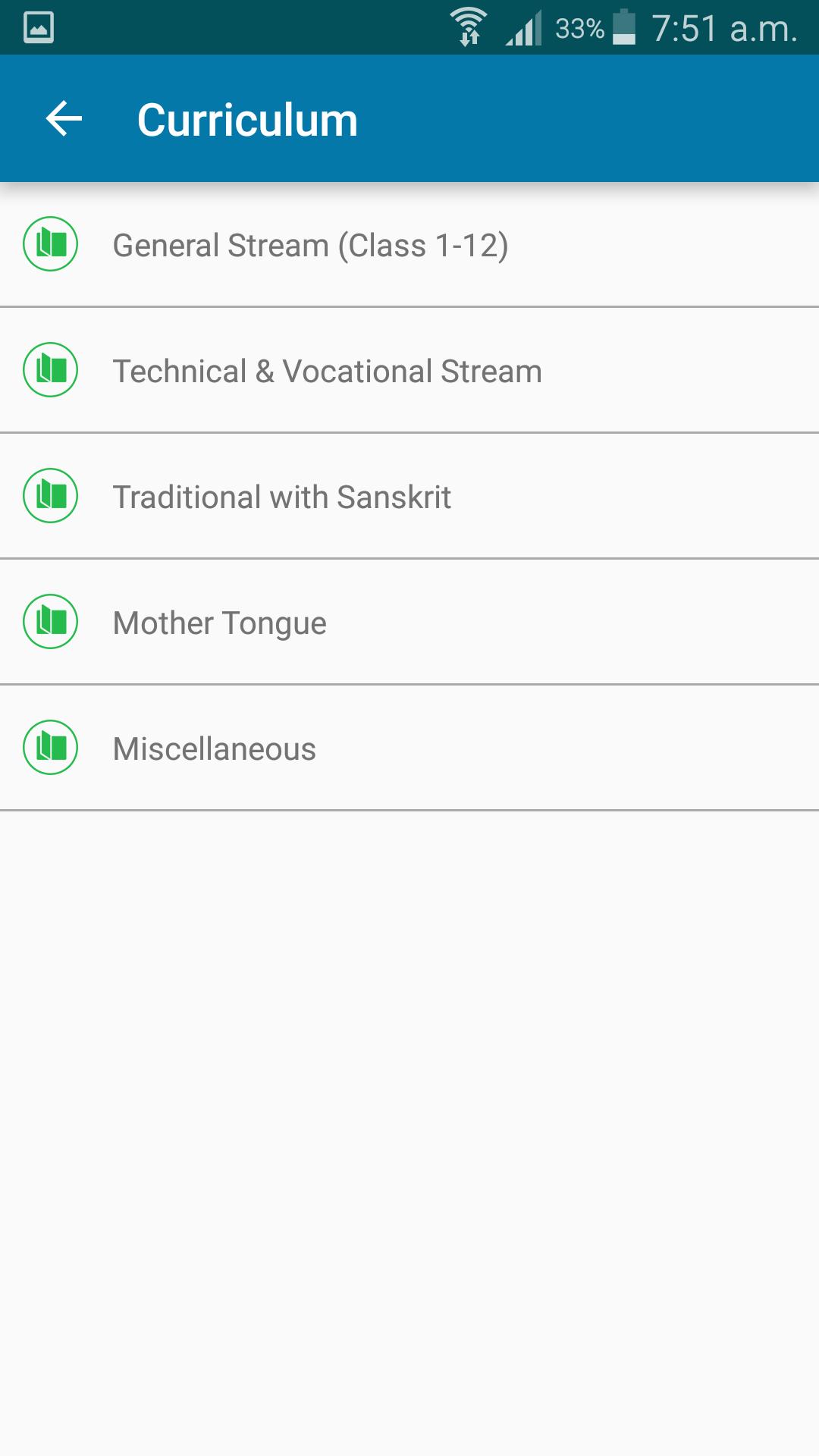The image is a colorful portrait-format screenshot from a mobile phone, captured at 7:51 AM. The phone's battery stands at 33%, with three out of four bars indicating a strong reception, and active data flow both in uploading and downloading. The screenshot prominently displays a section titled "Curriculum," which appears to be an interface from an educational app. The "Curriculum" heading is set against a blue banner, while the background below it is predominantly white or off-white with grayish text. Five distinct options are listed under the "Curriculum" category: "General Stream (Class 1-12)," "Technical and Vocational Stream," "Traditional with Sanskrit," "Mother Tongue," and "Miscellaneous." These options suggest various educational streams available within the app.